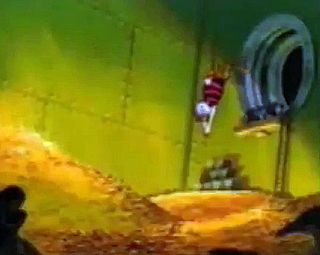The blurred, animated illustration depicts an interior scene resembling a green-tiled or metallic tank with sections woven together. On the right-hand side, a large grayish or silver circular opening leads to a platform accessible by ladder. From this platform, a figure, possibly a woman or animal, is diving headfirst into a pile of yellowish-brown material below. The diver, with red and white striped clothing and possibly a white hat or swimming cap, appears to be in mid-dive with arms extended forward. The figure's attire might also include dark ears or glasses. The green and yellow-toned walls of the structure feature a chartreuse hue, and there is an indistinct, silhouetted figure or shape in the lower left-hand corner. The pile at the bottom could be dust, gold, grain, or straw.